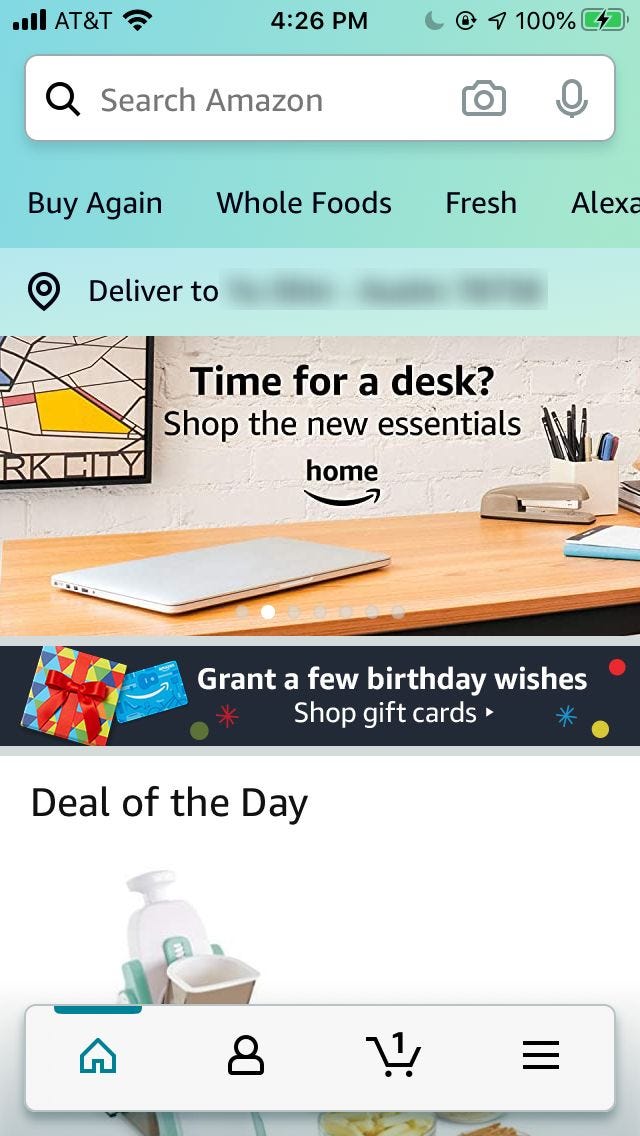The image is a screenshot of the Amazon application displayed on a mobile device. The device shows a full-strength carrier signal with four bars, provided by AT&T, with Wi-Fi enabled. The time is indicated as 4:26 PM. In the notification bar, there are icons for a crescent moon (possibly indicating Do Not Disturb mode), a lock with an arrow (suggesting orientation lock), and a location indicator showing that location services are enabled. The battery icon shows a 100% charge, and the device is currently charging.

At the top of the Amazon app interface, there's a white search bar containing the text "Search Amazon," accompanied by camera and microphone icons. Below the search bar, there are navigation options labeled "Buy Again," "Whole Foods," "Fresh," and "Alexa." The page indicates delivery details with a "Deliver to" section.

An advertisement banner on the screen reads "Time for a desk - Shop the new essentials - Amazon Home," featuring images of a laptop, a desk, a white container holding pens, pencils, and sharpies, a beige stapler, and artwork depicting New York City. Additionally, there is a colorful banner in blue, yellow, and red that says, "Grant a few birthday wishes - Shop gift cards." A section labeled "Deal of the Day" is also visible.